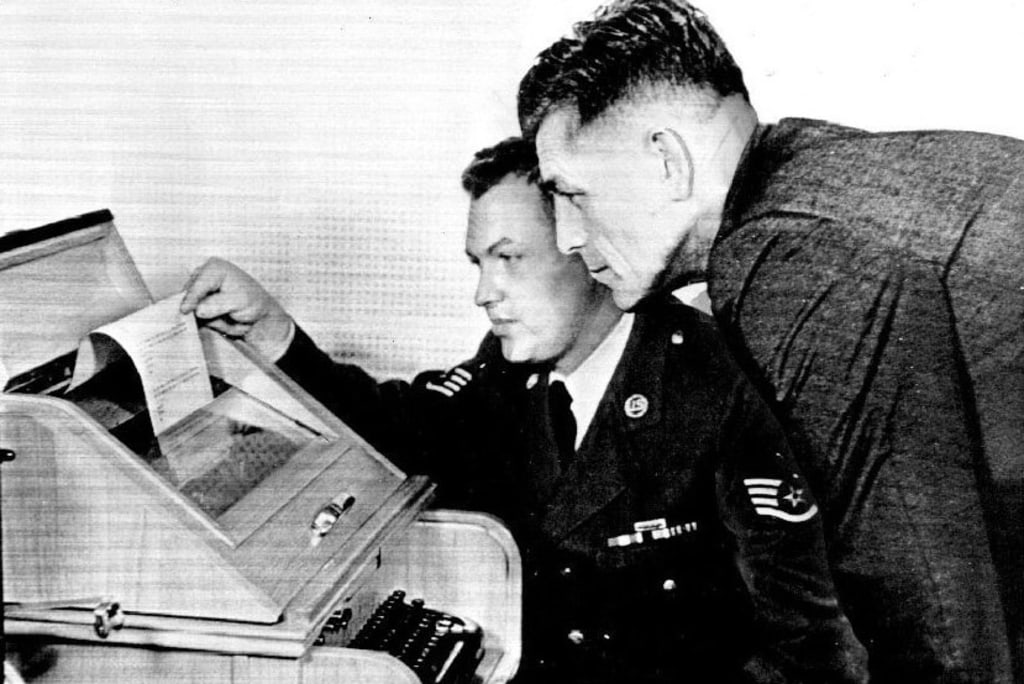This detailed description of a black-and-white vintage photograph from the 1930s or 1940s features two military officers engaged with an early communication device, possibly a telegraph machine. Both men are middle-aged with short, dark hair stylishly combed, the officer on the right is bending over from the waist, his left profile visible as he examines the machine. The man behind, seated, is clad in a dark military uniform complete with stripes on the arm, a white shirt, and a black tie. He holds a piece of paper emerging from the machine, which resembles a triangular wooden typewriter with a clear glass screen and keyboard below. The background presents a grey, textured wall, highlighting the striking contrast of this vintage scene.